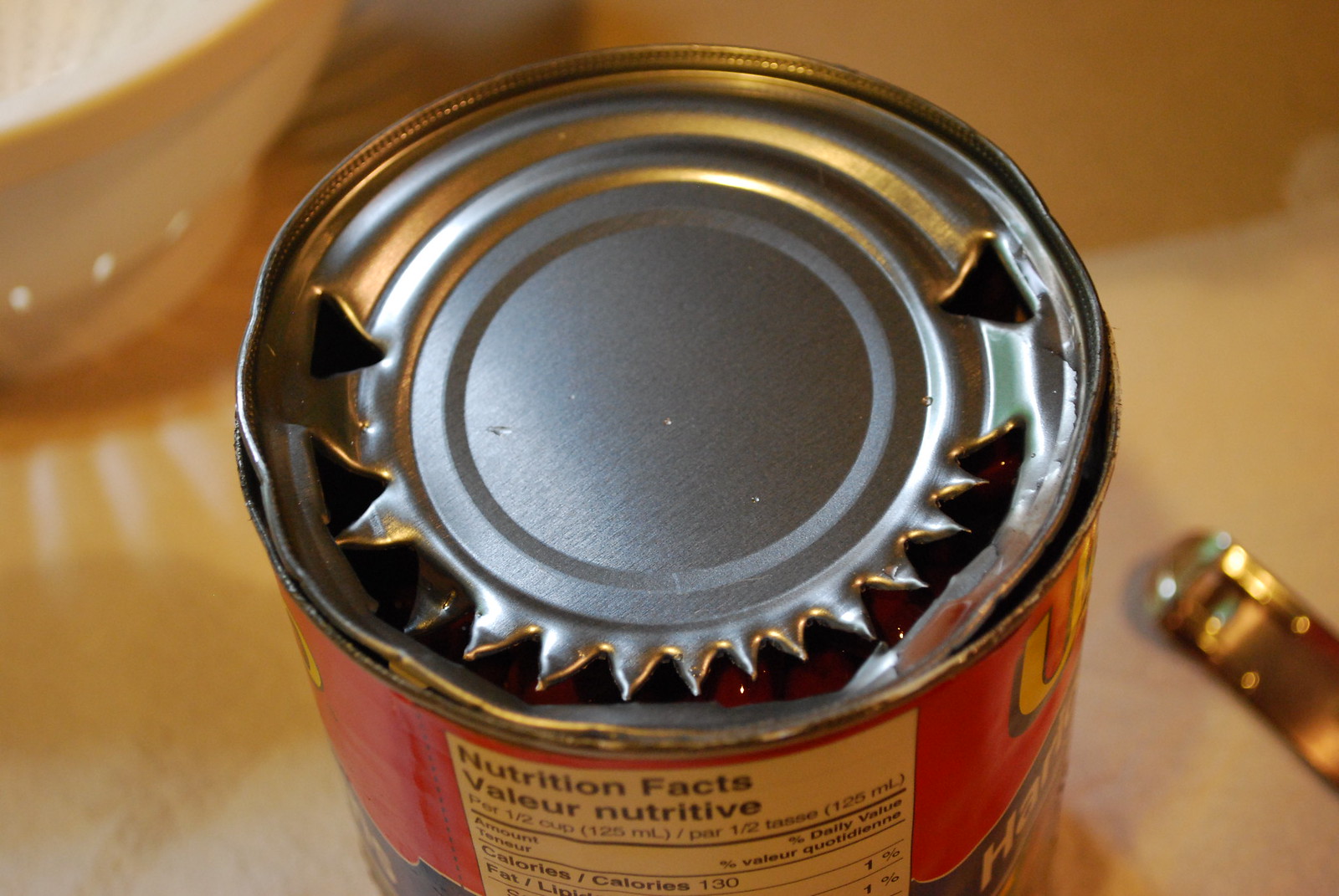The image depicts a close-up view of a partially opened tin can, featuring jagged and sharp triangular cutouts along its top half and covering roughly half its circumference. The can has a vivid red and blue label adorned with foreign text, including phrases such as "velour in nutritive," and detailed nutrition facts in both English and another language. Visible text includes "per 1/2 cup (125 mL)," "Calories/Calories 130," and "Fat/Lip 1%." The can is surrounded by reflections from the light, emphasizing the metal's sheen. Positioned slightly above the lower right corner of the can rests an old-style metal can opener used to make the jagged incisions. The background is heavily blurred, displaying a creamy yellow light and a white bowl in the upper left corner against a surface that seems to resemble marble.